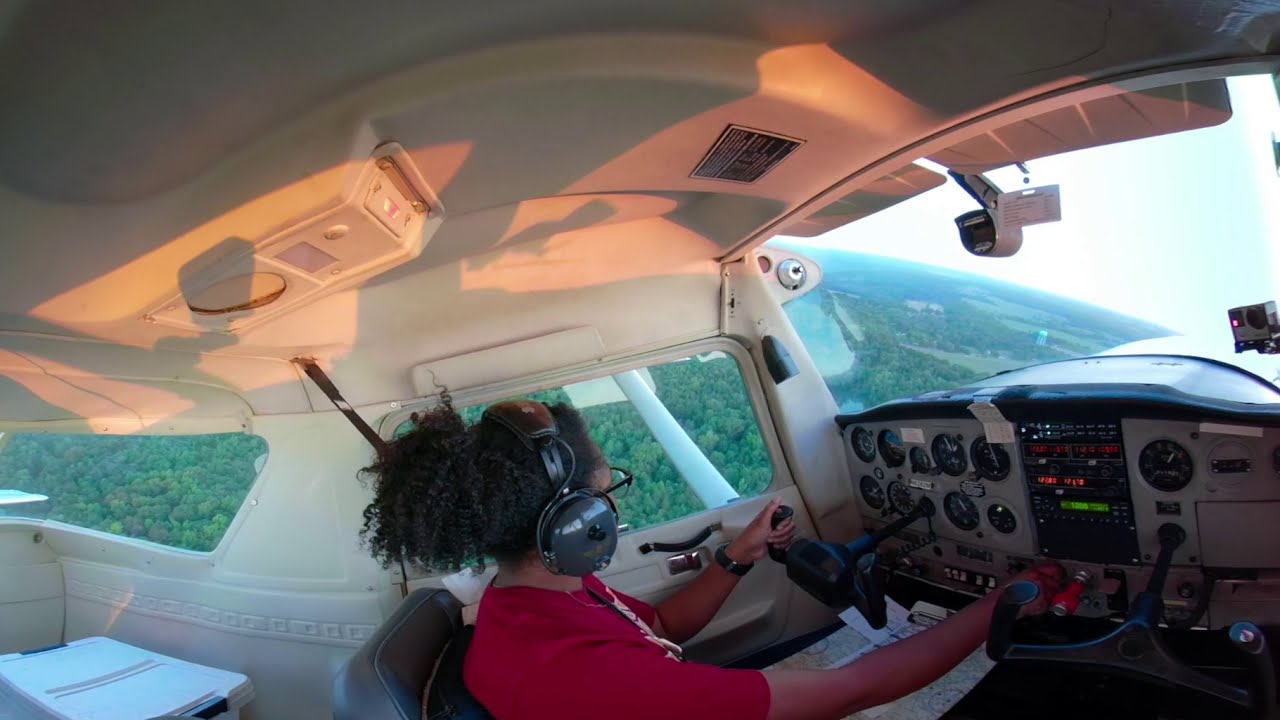The image captures Candice Dean, an African American woman, in the cockpit of a small airplane. Candice, wearing a red short-sleeved shirt, black-rimmed glasses, and large dark gray headphones over her ears, is at the center of the frame. Her thick, curly hair is pulled back into a frizzy ponytail. She holds the airplane's wheel with her left hand while her right hand is adjusting a button on the control panel. She is seated in a gray seat, with a white cooler situated just behind her. The cockpit's interior is light tan, featuring various dials, gadgets, and controls to her right. Sunlight with an orange hue reflects off the top of the image, suggesting it may be early morning or late afternoon. Through two side windows and the front window, a lush, green landscape peppered with airplanes, trees, and open spaces can be seen, indicating that the plane is flying high above the ground.